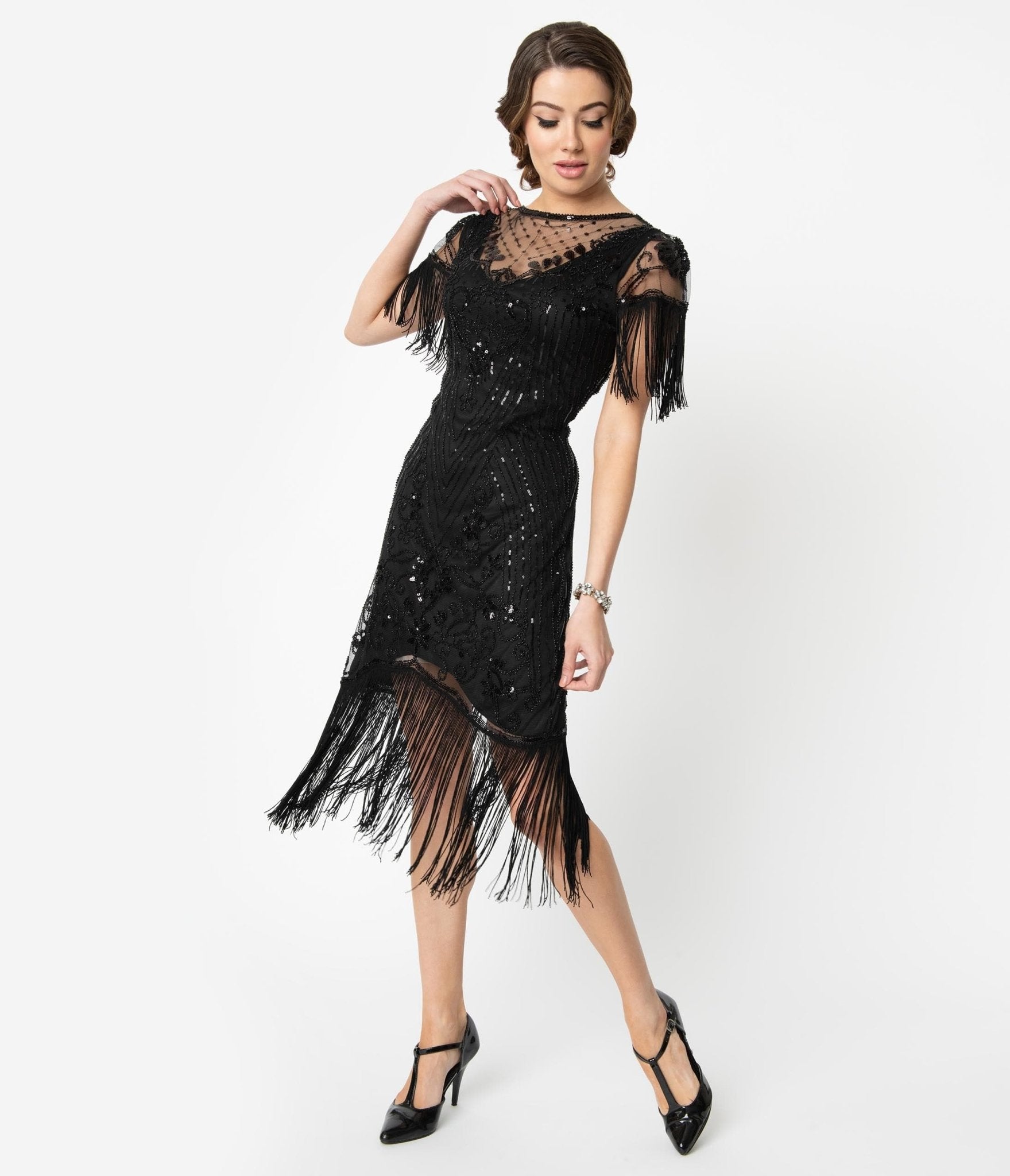The photograph features a woman in a stylish, 1920s-inspired black dress adorned with elaborate details. She stands against a plain white background and floor, her body oriented towards the camera while her head faces down towards her left foot, which is pointed and slightly bent. Her dark brown hair is elegantly pulled back into an updo, highlighting her long eyelashes and sophisticated makeup.

Her dress is characterized by a shimmering, fitted design that comes down to just above her knee before transitioning into a long, black fringe at the bottom. The dress has a V-neckline with sheer material extending up to her neck, and quarter-length sleeves that are transparent and adorned with fringe. The dress's top features intricate lace details, contributing to its glamorous appearance.

Her right hand is bent upward, resting on her right shoulder, while her left arm hangs by her side, adorned with a sparkling diamond bracelet. She completes the ensemble with black pointy heels that have T-straps and are about two inches in height. The overall composition of her pose and attire evokes the elegance and flair of the Roaring Twenties.